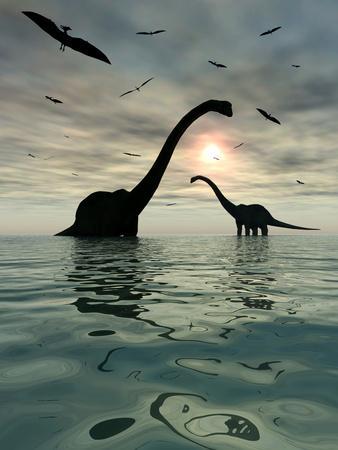In this evocative digital drawing, two majestic Diplodocus dinosaurs stand in serene, deep grayish-blue waters, their silhouettes set against a dramatic backdrop of a sunset sky with dark gray, pink, and yellow clouds. The foreground diplodocus on the left faces right, while the one in the background on the right looks left, creating a sense of balance and symmetry in the composition. Their long necks and small swan-like heads stretch out gracefully, their large, rounded bodies and elongated tails partially submerged in the shimmering, still water that reflects the dim sunshine breaking through the clouds. Above, a multitude of silhouetted pterodactyls fill the sky, with one particularly large bird dominating the foreground, enhancing the scene's prehistoric ambiance. The detailed ripples and reflections in the water add to the lifelike quality of this captivating image.